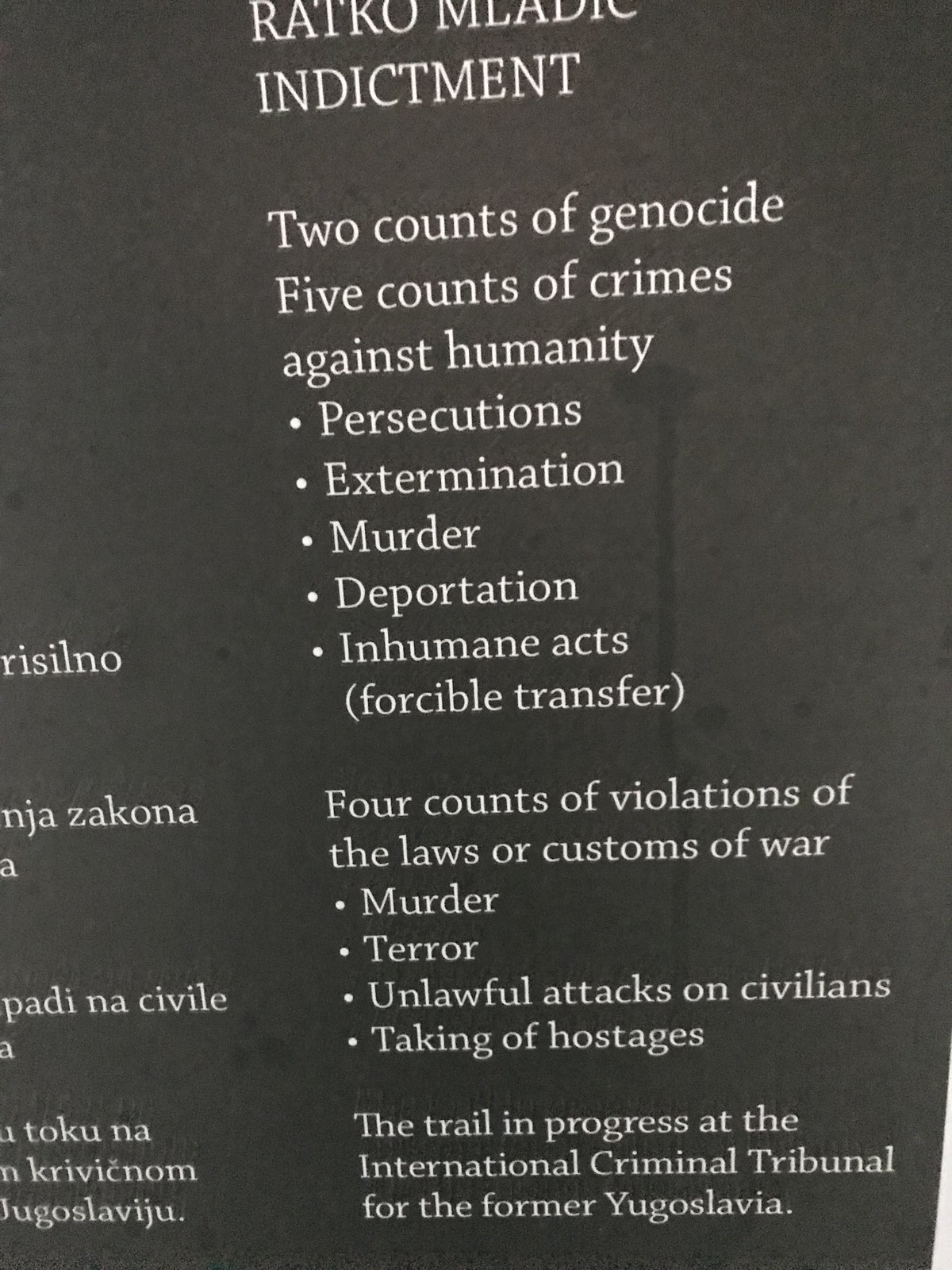The image features a portrait-oriented, black background with white text framed mostly in a central column and partially visible text in a foreign language on the bottom left. At the top, bold letters spell out "RATCO MELODIC" though the final letters are cut off. Below the heading, the text reads "Indictment" followed by detailed charges: "Two counts of genocide," "Five counts of crimes against humanity," with bullet points listing "Persecutions, Extermination, Murder, Deportation, Inhumane acts (Forcible transfer)." Further down, it states "Four counts of violations of laws or customs of war," with bullet points "Murder, Terror, Unlawful attacks on civilians, Taking of hostages." The bottom part of the image concludes with the statement "The trial in progress at the International Criminal Tribunal for the former Yugoslavia."